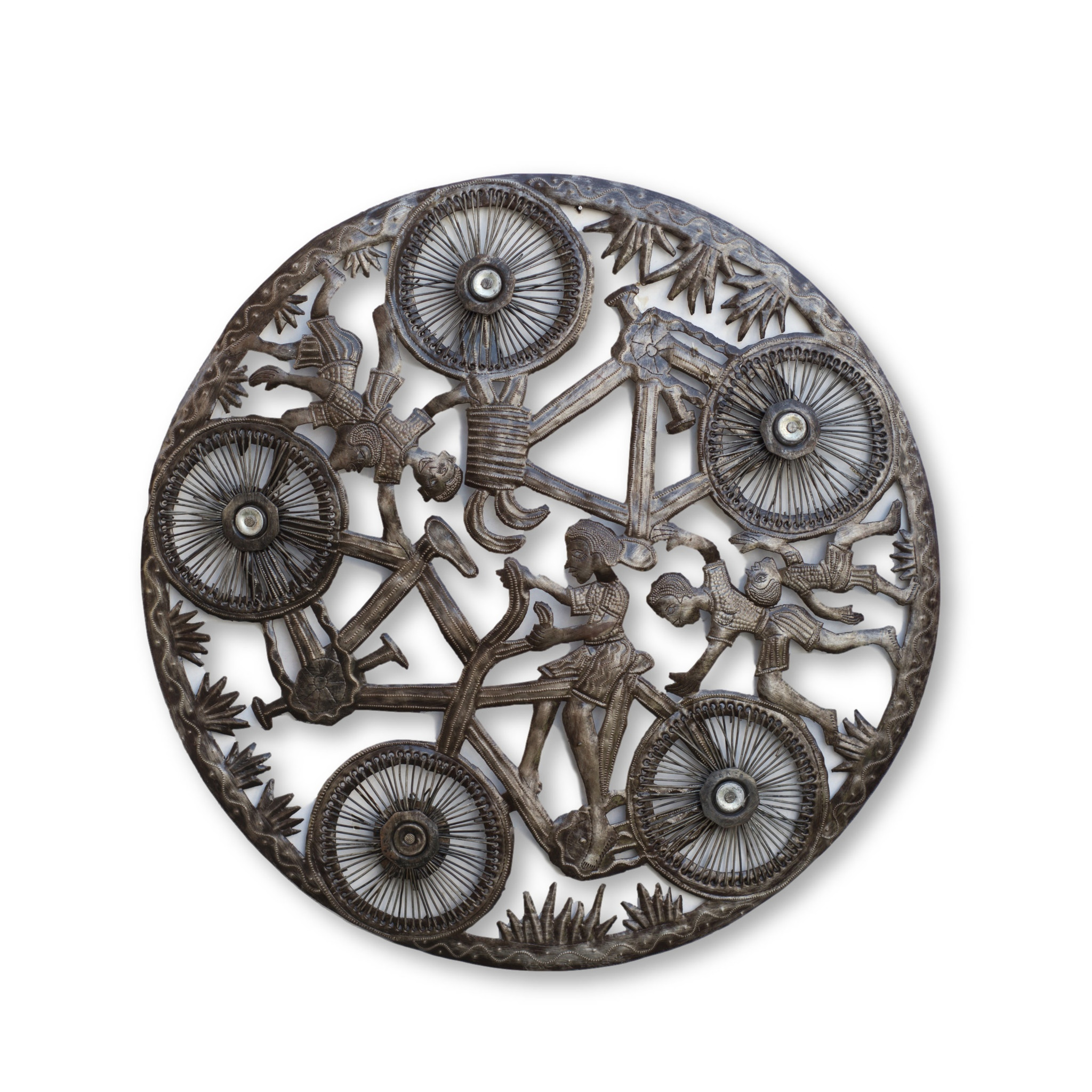This image depicts a circular artifact, seemingly made of a brass or bronze-like material, placed against a white background, giving it an isolated appearance. The object is intricately designed with a blend of artistic and mechanical elements. On the outer rim, there are spiral patterns adorned with dots and grass-like motifs emerging from the border. The center of the artifact features three bicycles, the wheels of which align with the outer edge, indicating a clockwise rotation. The riders, including adult and child figures, are positioned towards the inner part of the circle. The inner rim also exhibits grass patterns intertwined with the bicycle wheels, combining elements of nature and human activity. This artifact, which appears to be a carved medallion, showcases a unique fusion of native artwork and mechanical representation, emphasizing the imagery of cycling.